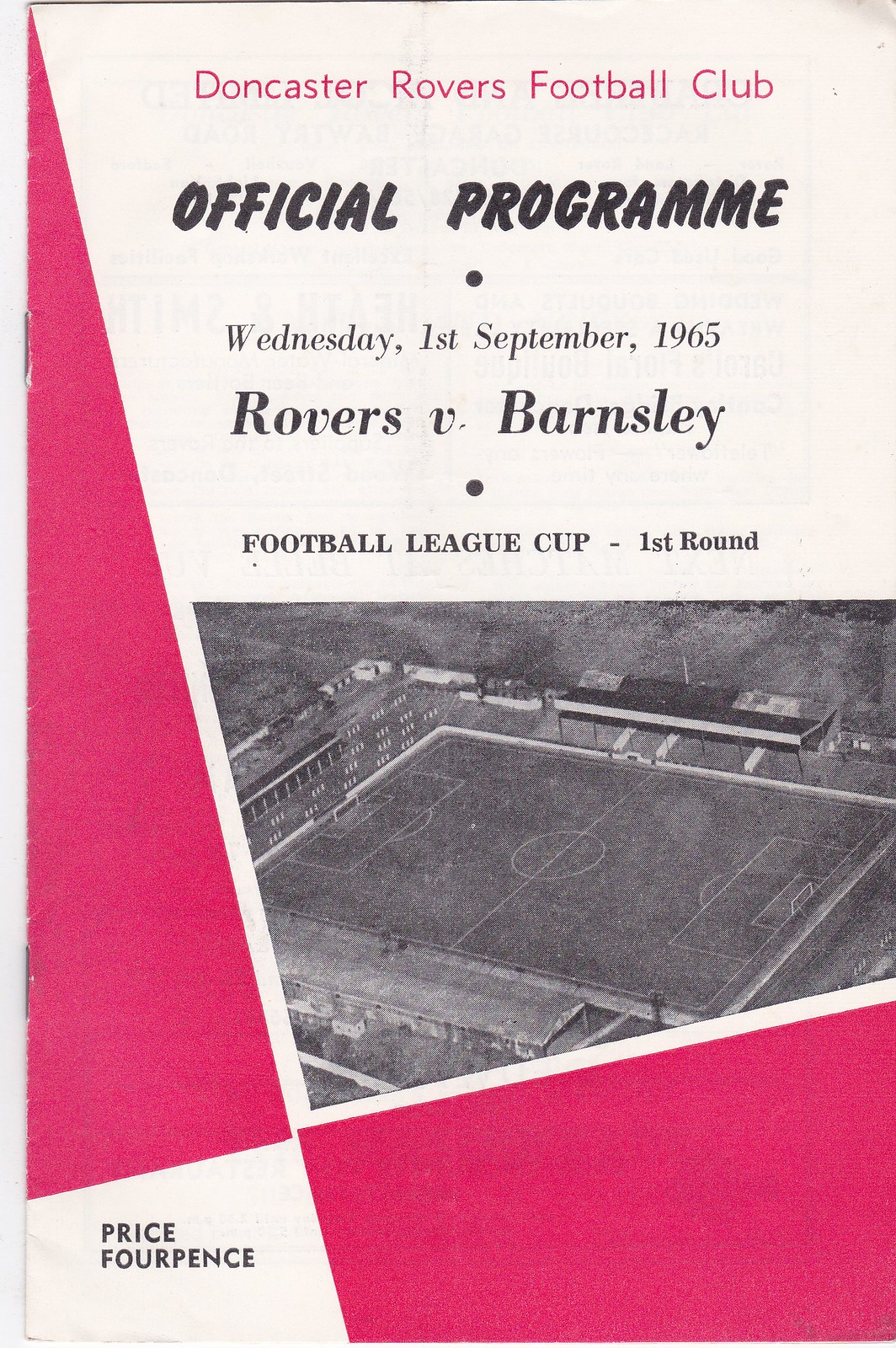This is a color photograph of the cover of a sports program for Doncaster Rovers Football Club, majority white with some red design elements. The title at the top reads "Doncaster Rovers Football Club" in vibrant red letters, and below it, "Official Program" appears in black text. Further down, the details of the event are stated as "Wednesday, 1st September, 1965, Rovers vs. Barnsley", with an additional note, "Football League Cup - 1st Round". At the bottom left corner, it mentions the price, "Price, 4 pence". The central feature of the cover is a black-and-white aerial photograph of a soccer field, with no players present. The image is of lower resolution, depicting a small, empty football stadium. The design is complemented by two geometric shapes, a red triangle and a trapezoid, which divide the cover into quadrants.